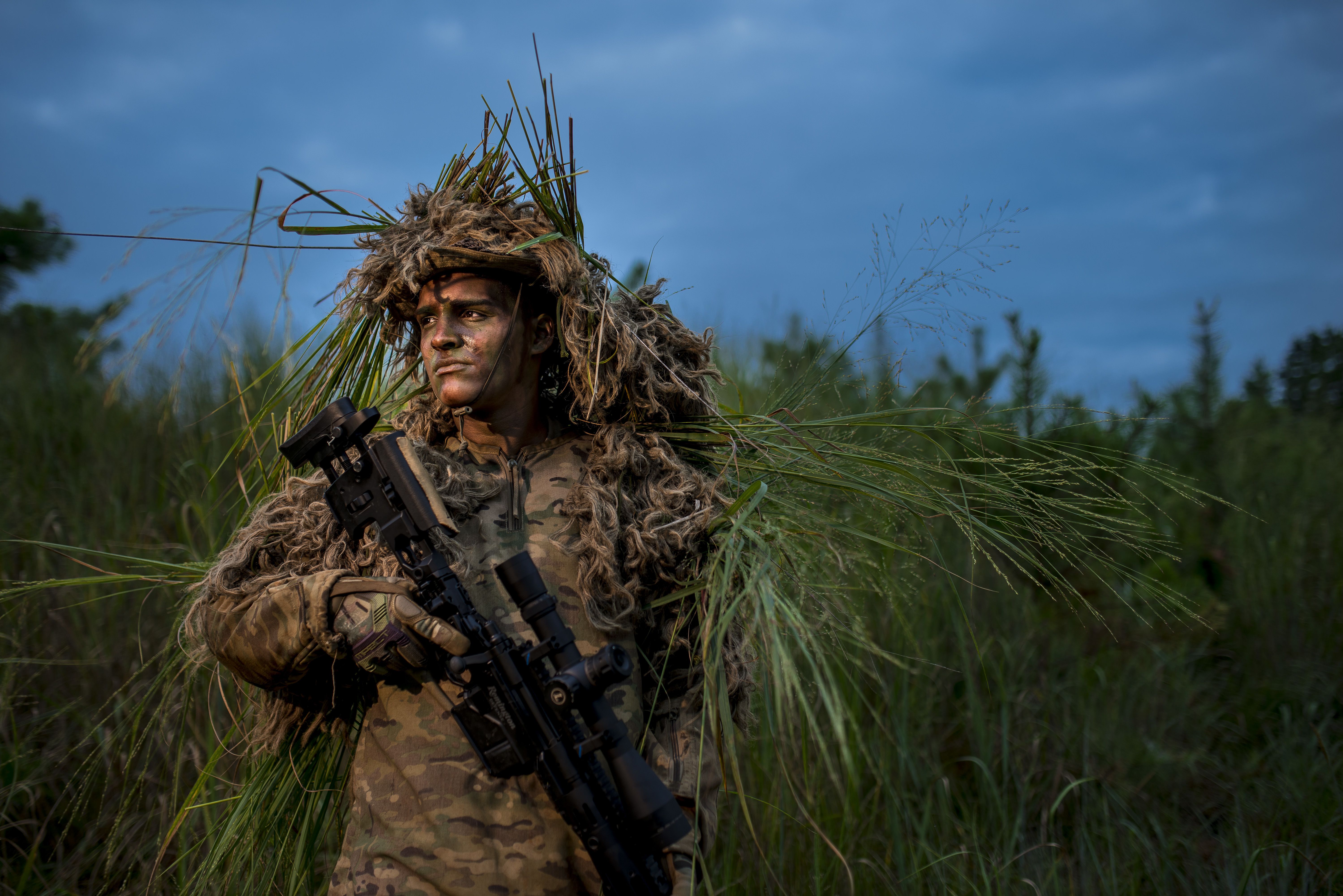The photograph captures a young, battle-worn man dressed in full camouflage attire, including gloves, and holding a large military-style weapon with a substantial scope. His tan skin is partially covered by light camouflage face paint or dirt, accentuating his tired and weary expression. His head is adorned with a mix of old plants and bushes, blending seamlessly with the surroundings. The background features vivid green tall grass and palm leaves, with the deep blue sky, possibly at dusk, enhancing the scene's dramatic tone. His intense, concerned gaze is fixed into the distance, emphasizing his vigilance. The composition's vivid colors and detailed textures create a striking contrast between the lush greenery and the twilight sky, emphasizing the man's integration into the natural environment as part of his camouflage.